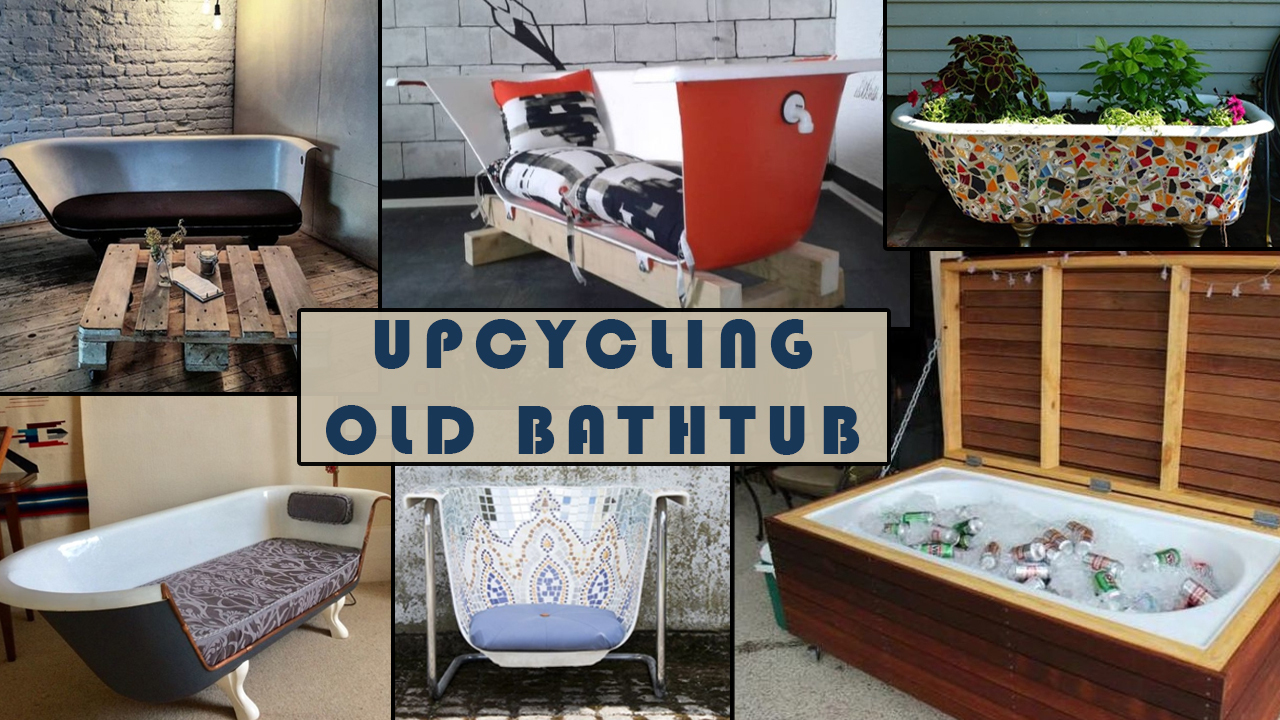This promotional brochure photo collage features six ingeniously upcycled cast-iron and porcelain bathtubs in various settings. Each image showcases a unique transformation of these classic fixtures into functional or decorative pieces. The focal point is a label reading "Upcycling Old Bathtubs."

1. **First Bathtub**: Positioned against a brick and wooden wall, this white bathtub with a black headrest has been cut in half. Its cozy setup includes a rustic pallet table adorned with a mason jar, a cup holding a small yellow flower, and a piece of paper, all resting on a wooden floor.

2. **Second Bathtub**: Painted red on the outside and white inside, this bathtub features a side cutout revealing its new use as a stylish indoor couch. It's furnished with plush red, white, and black pillows, supported by wooden beams along the bottom and sides.

3. **Third Bathtub**: This full, colorful bathtub is a garden centerpiece. Adorned with a mosaic of broken glass pieces in hues of red, maroon, cyan, orange, yellow, green, and dark blue, it is filled with soil and an array of plants, including a pink flower, a maroon-leafed plant, and a vibrant red flower.

4. **Fourth Bathtub**: Transformed into a vibrant seating arrangement, this half bathtub is fitted with a purple and maroon mattress and a glued-on gray headrest, creating a cozy indoor lounge area.

5. **Fifth Bathtub**: Shaped like a chair, this shorter bathtub features intricate embroidery and a crown-like back adorned with blue, golden, and white tiles arranged to mimic the sparkle of jewels, all supported by gray steel.

6. **Sixth Bathtub**: Repurposed as a cooler, this entire bathtub is encased within a wooden box. It is filled with ice and stocked with cans of soda and beer. The lid is reinforced with wooden crossbeams and is decorated with a string of lights.

In the center of the collage, a blue rectangular label reads “Upcycling Old Bathtubs,” tying together this creative and practical showcase of repurposed vintage bathtubs.